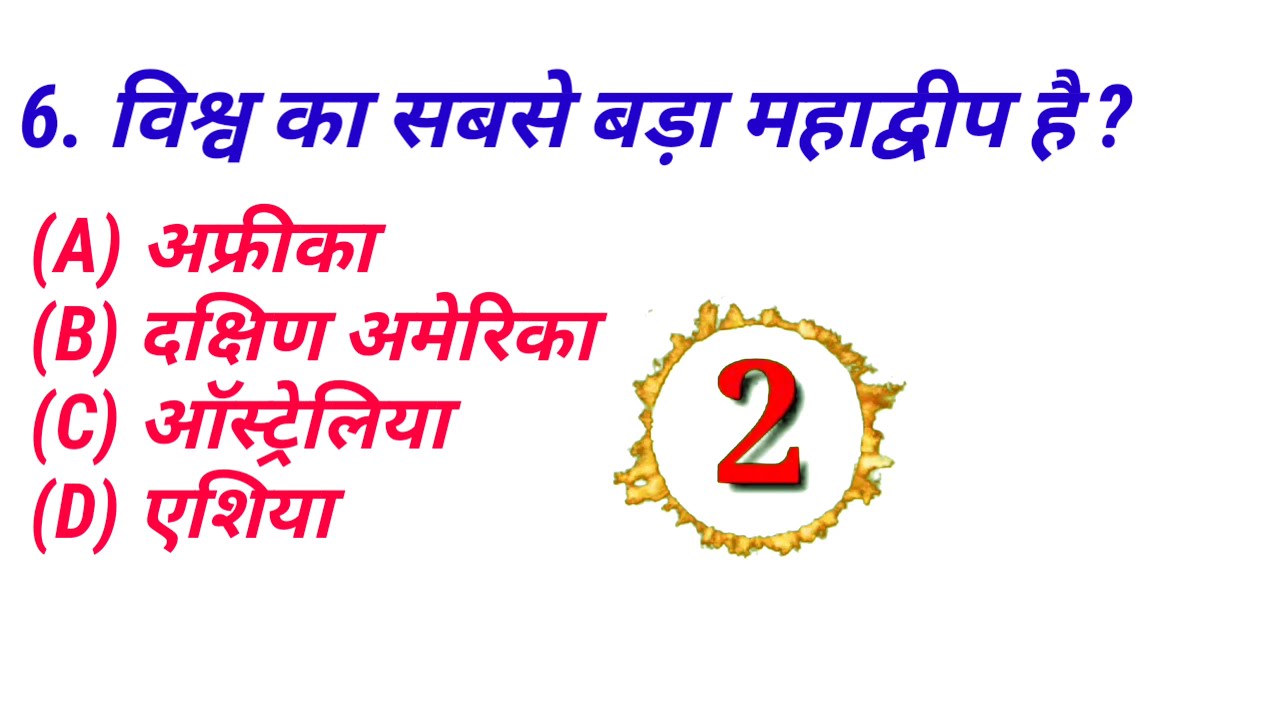The image features a white background with a structured layout that resembles an advertisement or educational content written in an Indian script. At the top, there is a numeral "6" followed by a period, and a question asked in blue font that ends with a question mark, indicating it’s likely a query or heading. Below this numeral "6," there are bullet points labeled A, B, C, and D, each accompanied by words in the same Indian script, indicative of multiple-choice options. Each bullet point ends with a character resembling 'T'. To the right of these options, prominently displayed, is a stylized circular emblem with a golden flaming border, encasing a large red numeral "2." This arrangement suggests organized information, possibly for an exam or questionnaire, with a visually striking element to the side.